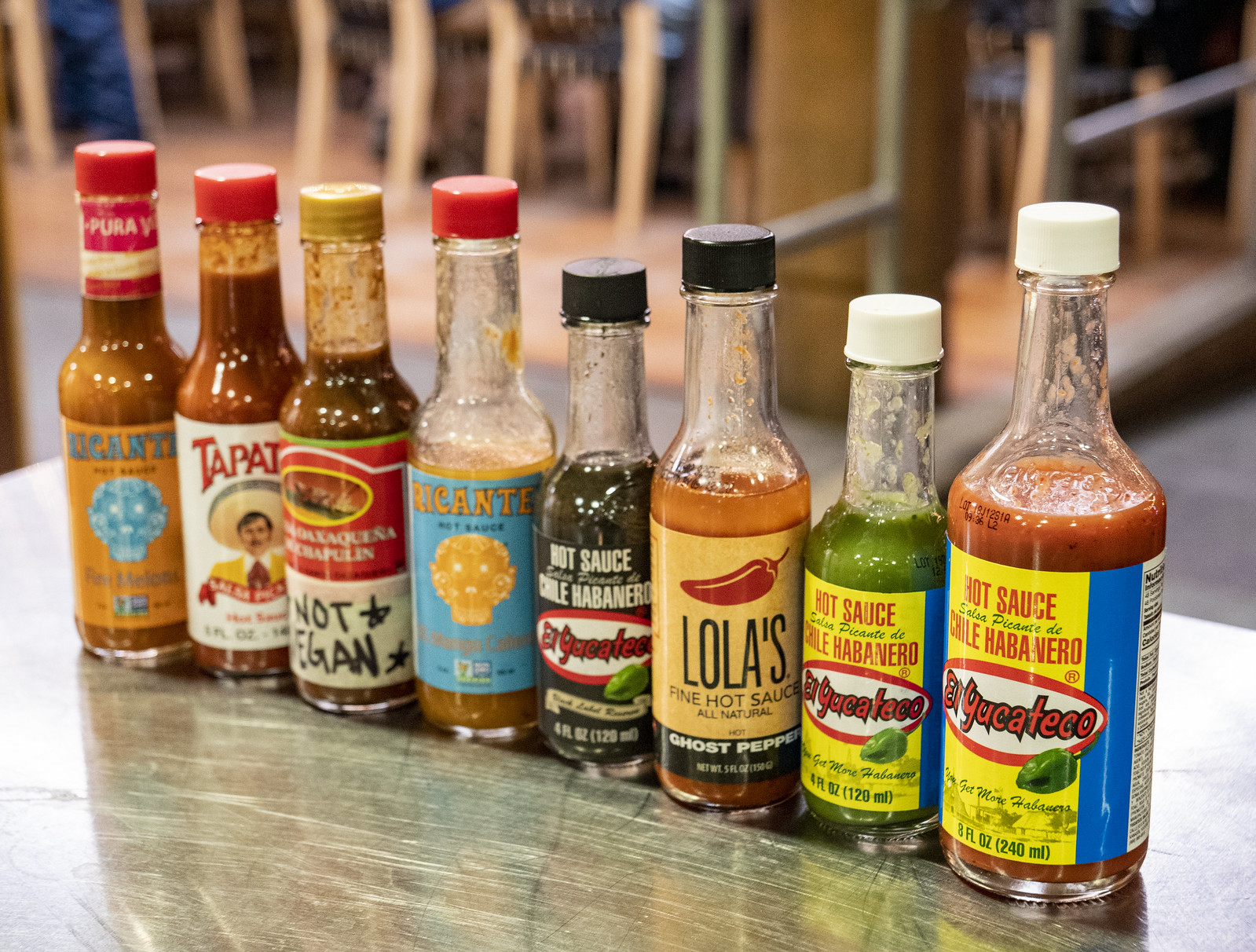In this color photograph, we see eight bottles of hot sauce arranged diagonally on a gray table, extending from the left center down towards the bottom right of the image. Each bottle is about four inches tall, with colorful labels and varying cap colors that include red, black, and green. In sharp focus, the hot sauces display an array of branding and design. From the left, the first bottle features a vibrant orange label with blue text and a red cap. Next is a bottle depicting a man in a sombrero, partially labeled with "T-A-P-A-T-O." The third bottle stands out with a red label prominently stating "not vegan." Following this is a bottle with blue and yellow elements and the partially visible text "Riconte," which is half-empty. Moving along, there's a black-labeled bottle inscribed with "El Uchico's Hot Sauce Chili Habanero," which is also half-empty. Then we see a bottle of Lola's Fine Hot Sauce sporting an all-natural ghost pepper label, followed by another "El Uchico's" bottle with a green label, and finally, a similar red-labeled bottle. The table catches some light from above, adding highlights to the scene. In the blurred background, chair legs and parts of tables hint at a restaurant setting, enhanced by a magenta tint to the overall image.